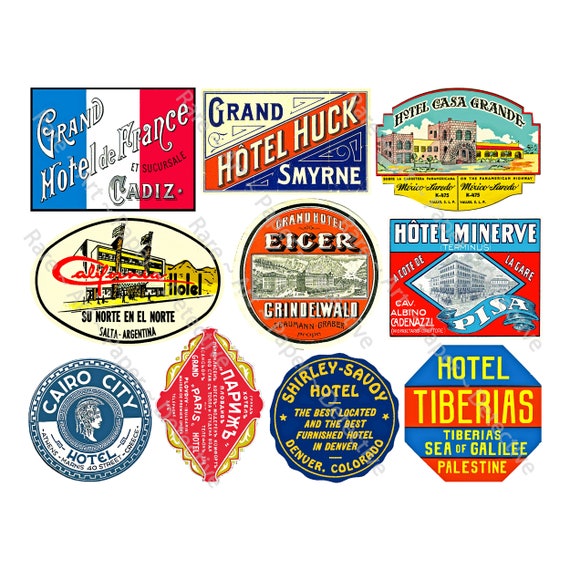The image showcases a vibrant collection of vintage hotel advertisements, arranged in a grid with three rows. Each of the ten colorful and detailed logos represents a unique hotel, evocative of a bygone era of travel and adventure. 

In the top row, the first advertisement features the Grand Hotel de France in Cadiz, framed with blue, white, and red, resembling the French flag. Next to it is the Grand Hotel Huck in Smyrne, characterized by white, orange, and blue hues. Following that, the Hotel Casa Grande, themed around Mexico, displays a picture of a building.

The middle row begins with a circular logo for the Grand Hotel Aiger in Grindelwald, depicting a building within a circle. Adjacent is the California Hotel advertisement, which mentions "Su Norte" and "El Norte." Additionally, the center hosts the logo of the Hotel Minerva Terminus, adorned with red and blue text in a foreign language.

The bottom row starts with the Cairo City Hotel, featuring an image of an ancient soldier and details about its location in Athens and Greece on 40th Street. A diamond-shaped, foreign language hotel advertisement follows. The Shirley Savoy Hotel in Denver, Colorado, renowned as the best furnished hotel in the city, is next with a striking blue circle. The sequence concludes with an octagonal logo for the Hotel Tiberias near the Sea of Galilee, Palestine, displaying red and blue elements.

This assemblage of hotel tags not only showcases a variety of shapes—rectangular, circular, diamond, and octagonal—but also captures a lively blend of colors and international allure, reflecting a spirited age of exploration and hospitality.